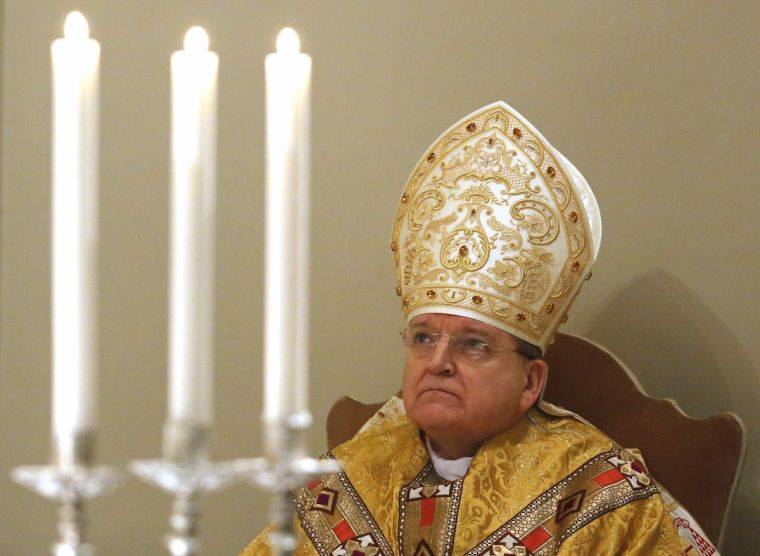The image features an elderly, white archbishop, around 60 to 70 years old, seated in a wooden chair with gold trim. He wears glasses and a mitre adorned with shades of gold and red rubies. His gold robe, decorated with intricate gold-bordered elements featuring black diamonds and red stripes, adds to his dignified appearance. He is looking upward with a serious expression, his shadow casting prominently against the beige wall behind him. In the foreground, three tall, lit candles in a silver-standing candelabra are out of focus, emphasizing the depth of the photograph. The light source comes from the top left, highlighting the archbishop and creating a shadow beneath and behind him. The serenity and solemnity of the scene showcase the archbishop's contemplative demeanor.